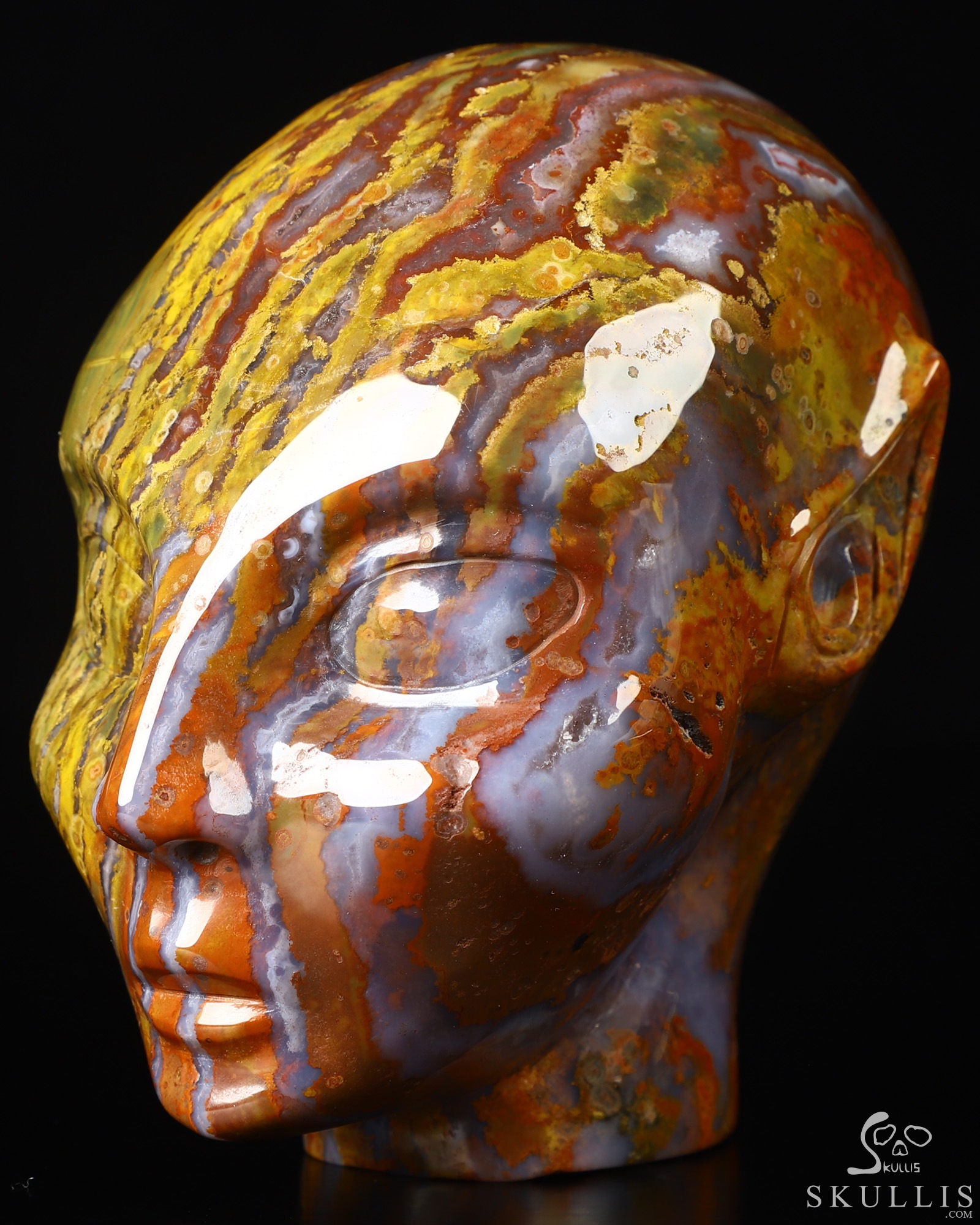The photograph showcases a striking marble head sculpture that resembles an alien or otherworldly figure. Set against a completely black background, the head fills the image, drawing all focus to its intricate details. The sculpture is depicted in a three-quarter view, highlighting its unusual shape with a pointed ear visible on one side. The face is eyeless, featuring empty eye sockets that enhance its eerie appearance. The alien head is predominantly red, accentuated by flowing rivers of gold color that cascade down its surface. The side of the face closest to the viewer has additional creamy bluish and pewter-colored streaks. In the lower right-hand corner of the image, a logo for Skullis.com can be seen, consisting of an outline of a skull with the name "Skullis" spelled out in modern, spaced lettering.